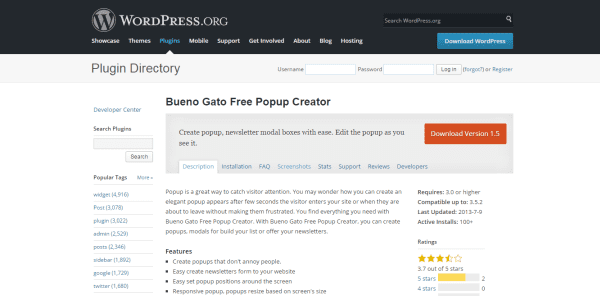The official website for the Bueno Gato free pop-up creator plugin on WordPress.org provides detailed information about its features and functionalities. The page prominently displays the plugin's name, "Bueno Gato Free Pop-Up Creator," along with the current version, which is 1.5. Below this, in smaller text, is additional information about the plugin.

The WordPress logo is prominently featured at the top in black, against a white and gray background. The WordPress icon is a gray circle with a blue "W" in the center. Beneath the logo, there is a navigation menu with various options, with the "Plugin Directory" section highlighted in blue, indicating the current section being viewed.

A light blue bar runs across the page with the text "Download WordPress" written in white. Further down, the page includes a comprehensive description of the Bueno Gato free pop-up creator plugin, detailing its capabilities and usage.

The focus of the page is the encouragement to download both the plugin (version 1.5) and WordPress itself, making it clear to users that the plugin can be easily integrated into their WordPress setup. The overall layout is clean and user-friendly, providing all necessary information at a glance.